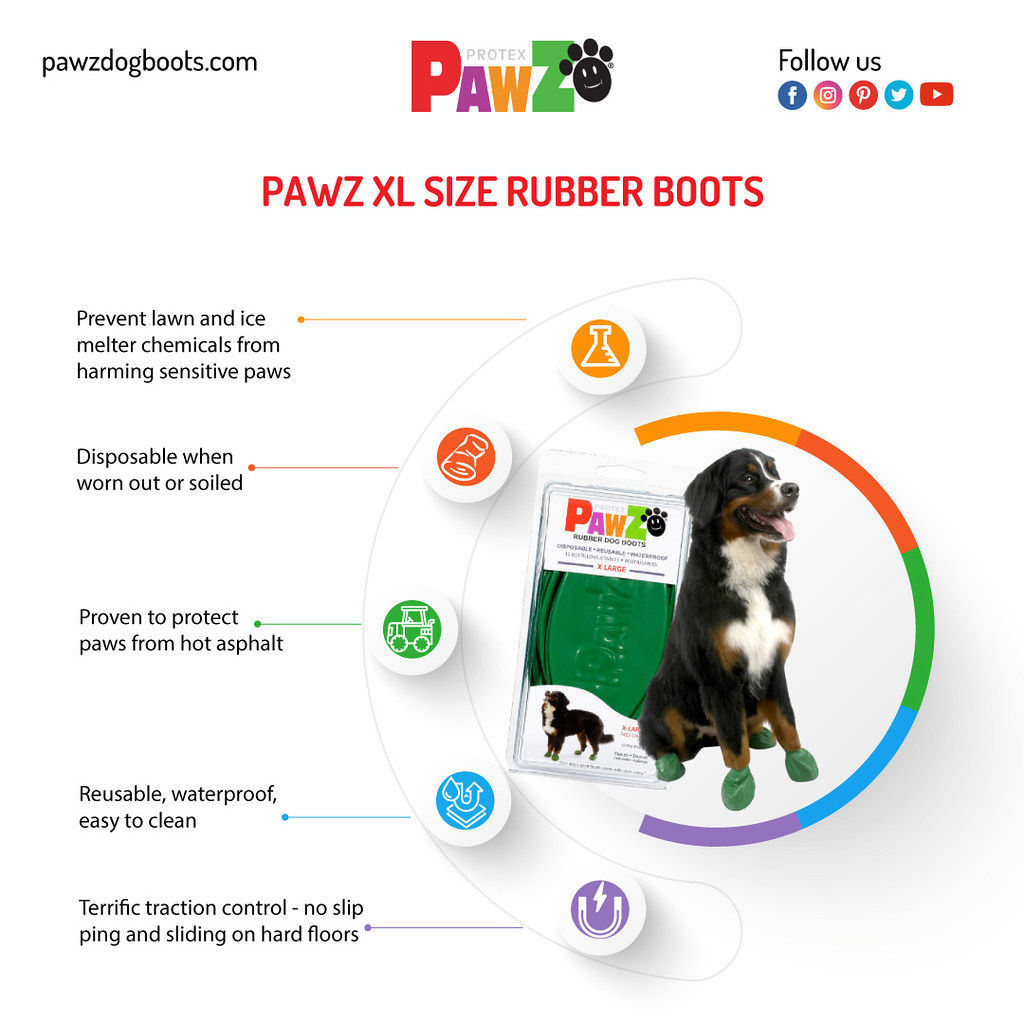This is an advertising poster for Pawz rubber boots for dogs, showcasing their extra-large size green boots. At the top left of the poster is the website "pawsdogboots.com" in dark black against a white background. Centrally placed at the top is the vibrant "Pawz" logo, with the letters colored in deep red, purple, yellow, and green, respectively. Next to the logo is a circular face icon with four ear-like protrusions, possibly representing a stylized dog, and to the right, social media icons for Facebook, email, Twitter, and forward, suggesting "follow us."

Beneath the logo, in red text, it reads "Pawz XL size rubber boots." Central to the poster is an image of a cheerful Shetland dog wearing the green Pawz boots, and behind the dog, there’s an image of the product’s packaging. To the left of the dog, detailed features of the boots are listed:
- Prevent lawn and ice melter chemicals from harming sensitive paws.
- Disposable when worn out or soiled.
- Proven to protect paws from hot asphalt.
- Reusable, waterproof, and easy to clean.
- Terrific traction control, ensuring no slipping and sliding on hard floors.

This comprehensive and educational poster advertises the versatile and protective Pawz rubber boots designed specifically for dogs.